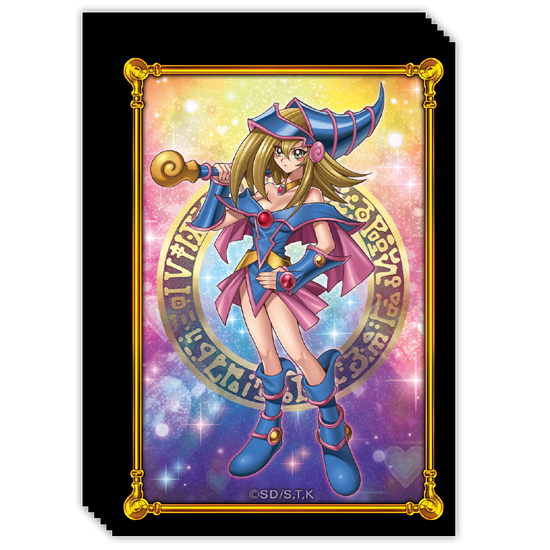The image depicts a vertical black rectangular card, characteristic of a Yu-Gi-Oh! dark magical card, with intricate ridges on the top right and bottom left corners as if torn. The card features a golden frame with rounded edges, slightly aligned to the right and downward, creating a more substantial black border on the top and left sides compared to the bottom and right. Inside this frame, an illustrated animated woman with brown hair stands confidently, her left hand on her hip while holding a staff or flag with a brown tip in her right hand. She wears a distinct blue, conical hat that curves upwards at the back, a blue top paired with a purple skirt, a matching purple cape, and large blue boots.

Behind her, a circular gold outline is inscribed with various symbols, adding a mystical aura to the illustration. The background within the frame is a starry gradient space scene, transitioning from yellow with white sparkling stars at the top, through pink in the middle, to a darker blue at the bottom. Small white dots resembling stars sprinkle throughout this celestial backdrop. Below the woman's feet is the text "SD/STK," seemingly part of the card's designation. The entire card is set against a white background, further emphasizing the dark, ornate design of the gaming card.